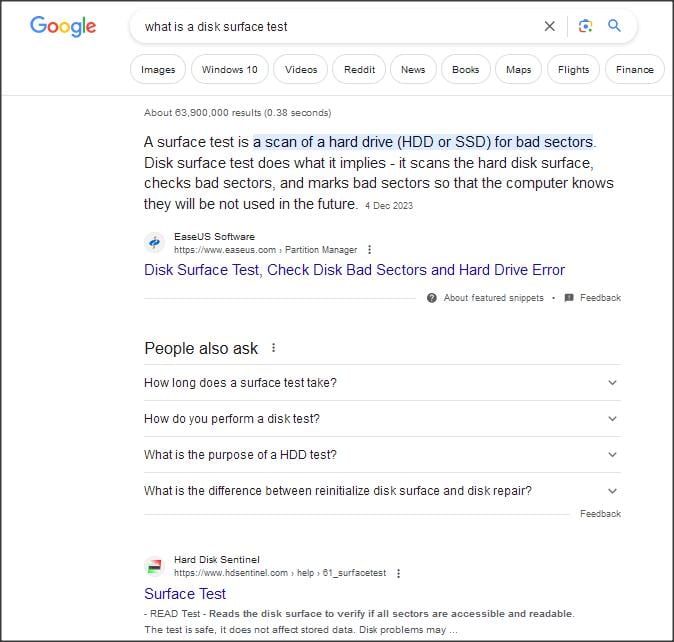A screenshot of a Google search results page displays information about a "disk surface test." The top result, sourced from EaseUS Software, dated December 4th, 2023, explains that a surface test scans a hard drive (HDD or SSD) for bad sectors, marking them so they are not used by the system in the future. Below this primary result, expandable pull-down menus reveal frequently asked questions related to the search query. These include: "How long does a surface test take?", "How do you perform a disk test?", "What is the purpose of an HDD test?", and "What is the difference between reinitializing disk surface and disk repair?". Further down the page, another link directs users to information from Hard Disk Sentinel, which also provides details about surface tests.